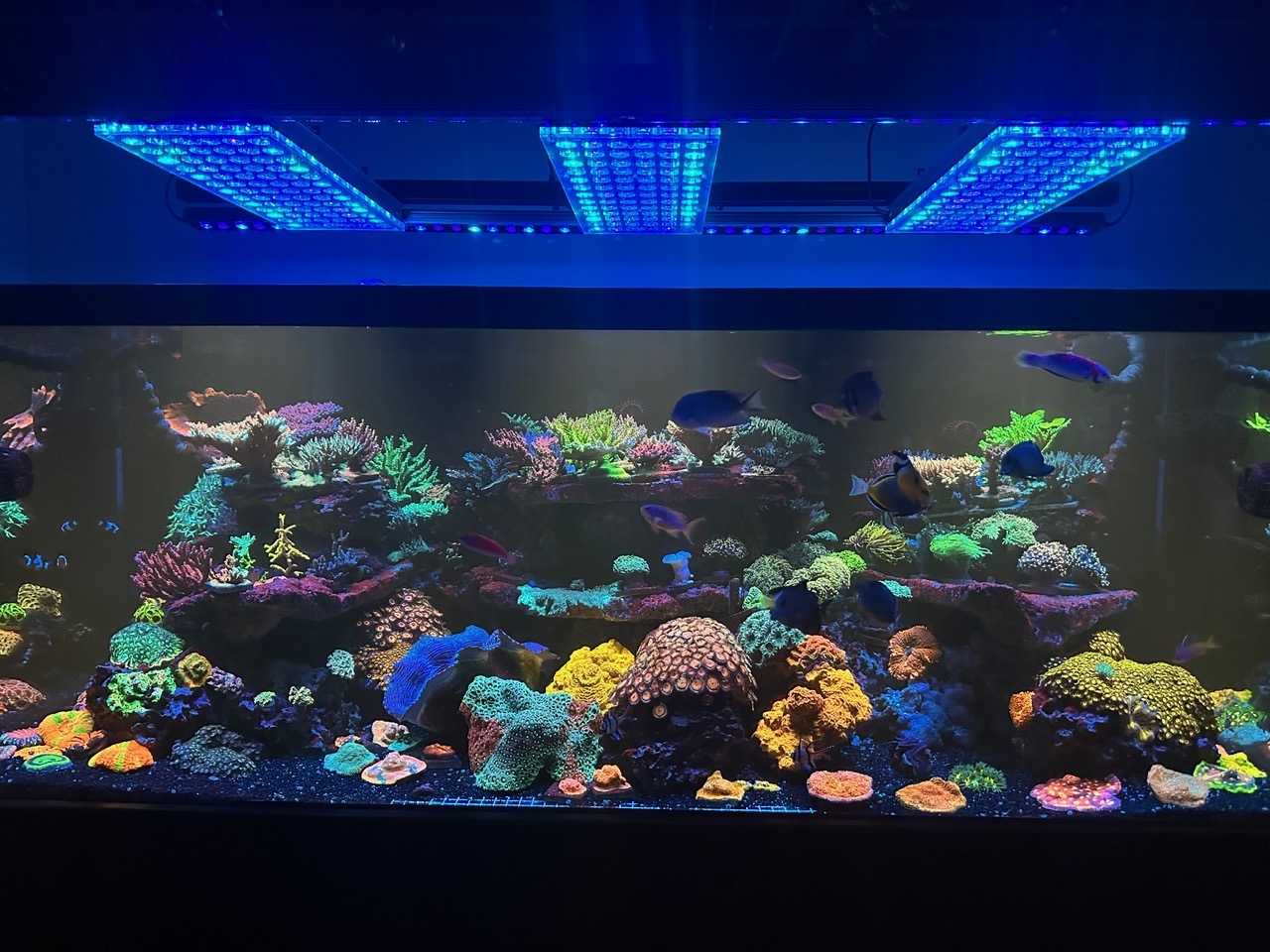The photograph captures a large, rectangular aquarium that occupies the central part of the image. The aquarium is illuminated by three rectangular panels on the ceiling, each equipped with tiny LED bulbs that bathe the scene in a fluorescent blue glow. Inside, a variety of colorful decorations, ranging from yellow and brown to green, pink, neon blue, and dark purple, mimic sea plankton and coral, creating a vibrant underwater landscape. A multitude of fish, primarily blue and pink, float gracefully amidst the ornaments. The overall setting exudes a vivid, aquatic ambiance, accentuated by the dynamic interplay of light and color.